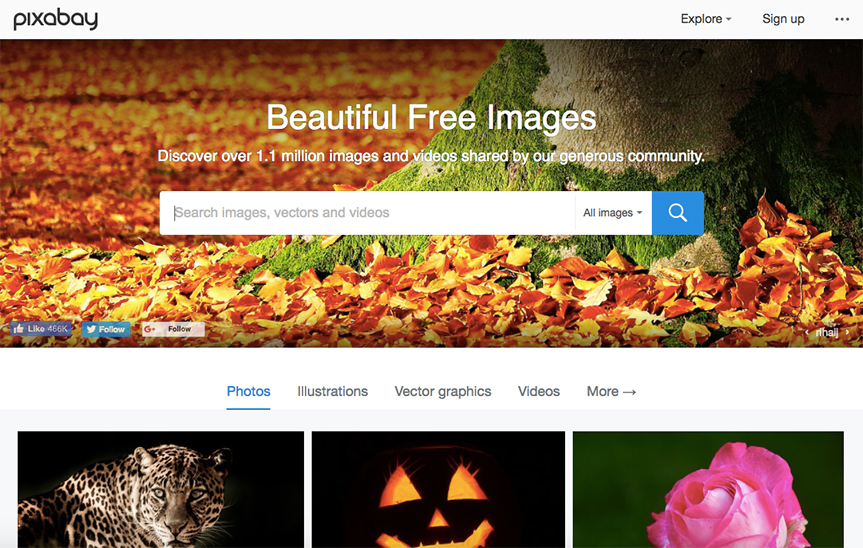The screenshot captures the homepage of the Pixabay website. In the top left corner, the "Pixabay" logo is prominently displayed. To the right of the logo, a drop-down menu labeled "Explore" with a downward-pointing arrow offers navigation options. Adjacent to this is the "Sign up" link for user registration, followed by three vertical dots likely leading to additional settings or options.

Below the header, a stunning image of a tree trunk surrounded by orangey-brown leaves dominates the scene. Overlaying this image in large white text are the words, "Beautiful free images." Beneath this, a subtitle reads, "Discover over 1.1 million images and videos shared by our generous community." 

Centered under this text is a search bar where users can input keywords to find specific images, vectors, or videos. A drop-down menu within the search bar allows for narrowing search results by category. A blue button on the right side of the search bar enables the search action.

On the left side of the screen, social media icons include a Facebook "Like" button with 466,000 likes, a "Tweet" button, and a Google Plus follow button.

Below the main features, a navigation bar indicates the current selection is "Photos," highlighted in blue. Alternative categories such as illustrations, vector graphics, videos, and more can also be selected. Three thumbnail images are displayed at the bottom: a leopard set against a black background, a black background with a Halloween lantern, and a beautiful horse with a green background.